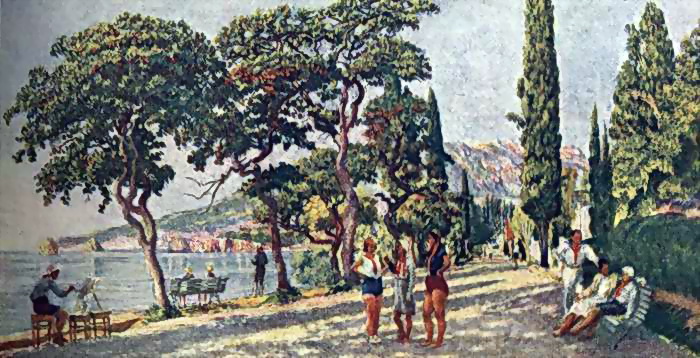This painting, titled "September Morning in Artec" by Ilya Mashkov and created in 1934, is an oil painting in a Russian Impressionist style. The scene, set in a lakeside park, exudes a 1950s Americana feel, conveyed through the clothing of the figures and the idyllic setting. 

In the foreground, three women stand on a wide gravel pathway. Two are dressed in 1950s-style swimsuit bottoms and tops, while the third wears a dress or beach blouse, engaged in conversation under the shade of squiggly-branched, manicured trees. To the right, a park bench hosts two seated individuals, while a man in a white outfit stands talking to them. Further, on the pathway that curves around the pond, a man is seated on the lower-left corner painting on an easel. Adjacent to him, another bench holds two more people, with someone standing nearby.

The background features a large blue sky with wisps of gray amidst towering trees and cypress, leading to a mountain or tall hill and clusters of distant buildings on the shoreline. The scene is rich in detail, capturing the leisurely atmosphere of a serene lakeside park.